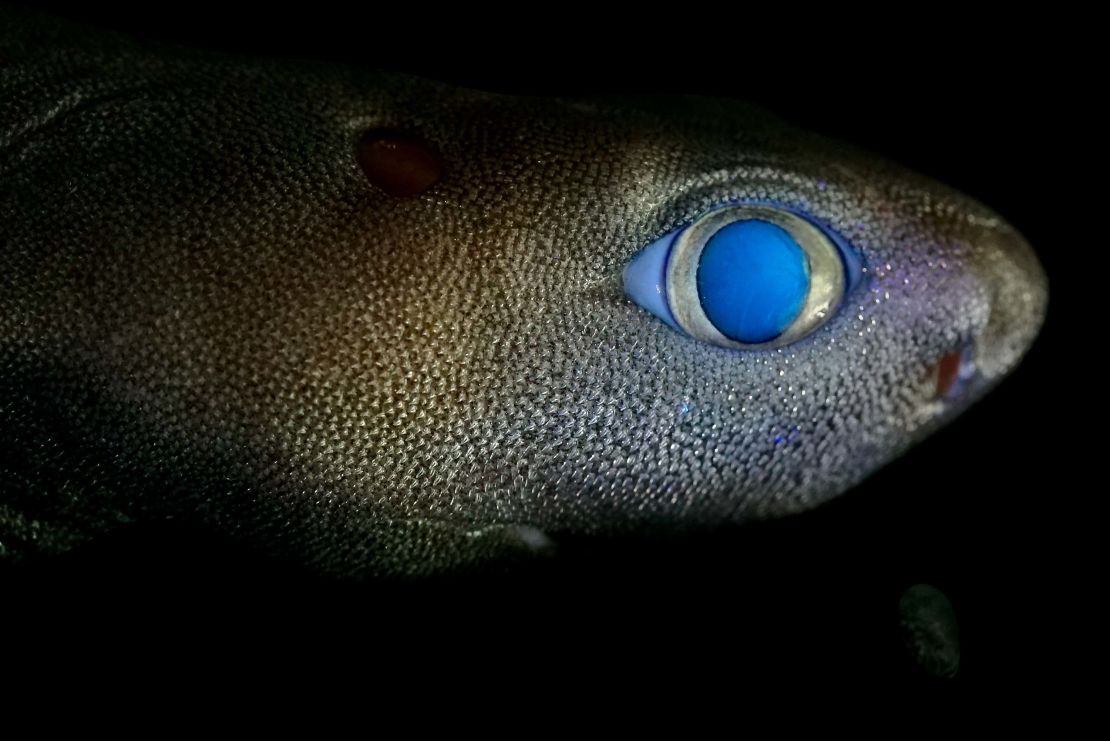This striking photograph captures a solitary fish set against a pitch-black background, creating a dramatic contrast that highlights the fish's features. The image showcases the fish from its face through most of its silvery-gray, brown-tinged body. The centerpiece of the image is the fish's prominent eye, which demands attention. The large eye features a deep blue central circle, encircled by a silvery, pearlescent ring that gives way to a lighter blue halo. Although the fish's mouth is somewhat indistinct, it is suggested by a line. Just above this line, a small, dark reddish mark adds a touch of intrigue to the fish's appearance.